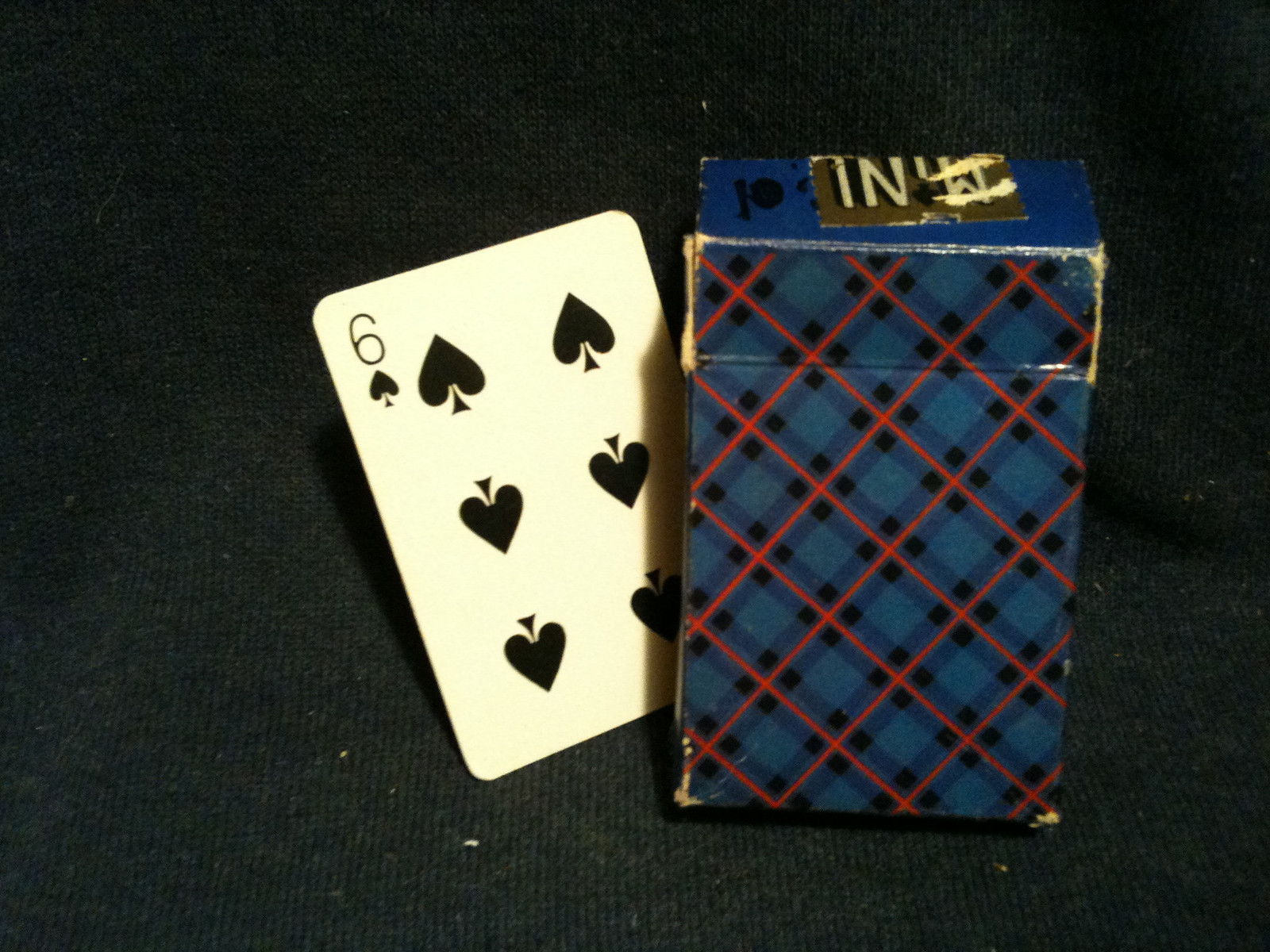The photograph features a predominantly black tablecloth, which serves as the backdrop for the subjects in the image. Central to the composition, slightly offset to the left, is a six of spades playing card. The card is not lying flat; instead, it is propped up slightly, suggesting it is being held by an unseen object or force. Positioned in front of the card, marginally to the right and obscuring the bottom right corner of the card, is the deck's box. The box stands upright and showcases a distinctive grid-like pattern. The grid is characterized by red intersecting lines overlaid on a blue background that also features grid elements. 

The box exhibits signs of wear, especially noticeable at the top where the colors have faded, revealing brown spots. This top section differs in color, presenting a more vivid shade of blue compared to the rest of the box. Adorning the center of the top is a rectangular sticker, yellowish-brown in hue, marked with heavily worn letters that render the text illegible. Additionally, there is a partially discernible black logo located at the top-left corner of the box.